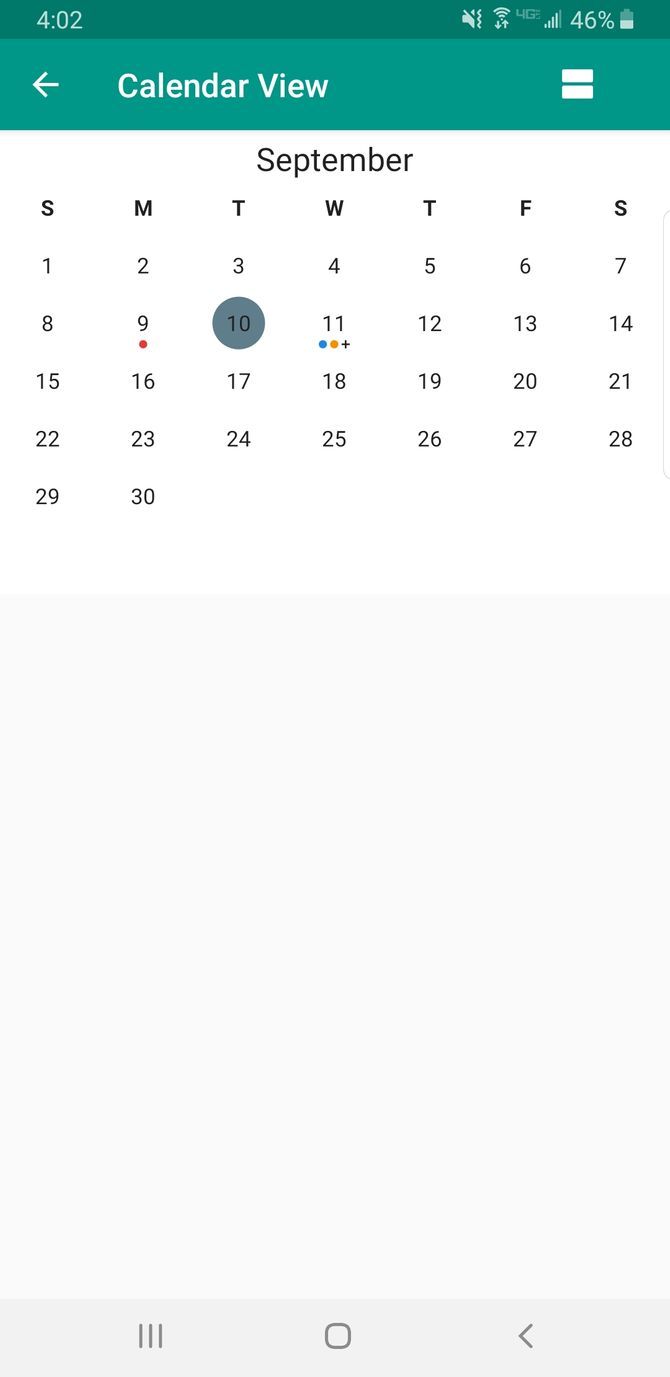The image depicts a screenshot from a smartphone's calendar application. In the upper left-hand corner, the time displayed is 4:02. On the upper right-hand side, the battery level is shown at 46%. The calendar is open in "calendar view" mode, as indicated below the status bar information. The currently displayed month is September, with the days of the week starting from Sunday on the left to Saturday on the right.

The calendar shows all 30 days of September, starting with Sunday the 1st and ending on Monday the 30th. The date highlighted, marked with a gray circle, is Tuesday, September 10th. Additionally, there is a red dot below the number 9, indicating an event on that date, and the number 11 features a blue and yellow dot with a plus sign, suggesting another event or reminder.

At the bottom of the screenshot, three navigation buttons are visible: a three-lined menu button, a home button in the center, and a back arrow button on the right.